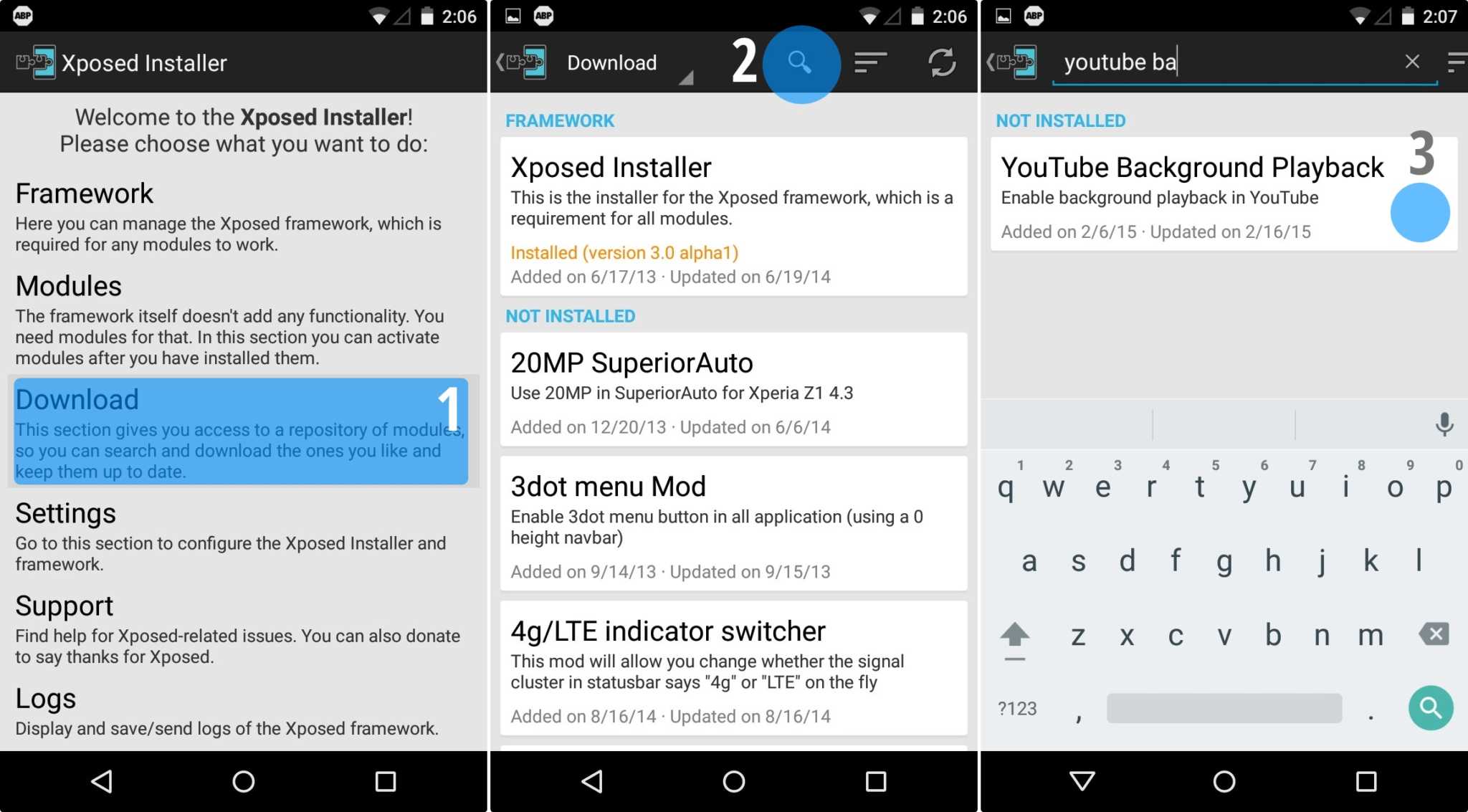This screenshot appears to be taken from a tablet or smartphone, as indicated by the presence of the familiar back and home buttons at the bottom. The image is divided into three columns, each containing distinct sets of information. The first column is labeled "Xposed Installer" with a black background and includes subsections named Framework, Modules, Download, Settings, Support, and Logs. The second column, also with a black background, is labeled "Download" and features entries such as Exposed Installer, 20MP Superior Auto, 3.MenuMod, and 4G LTE Indicator, each with accompanying descriptions. The third column, again with a black background, is titled "YouTube BA," and lists "YouTube Background Playback" as a primary entry, followed by what appears to be a QWERTY keyboard overlay. It seems that these columns showcase different types of software or modules related to the Xposed Framework, downloads, and YouTube functionalities, possibly resulting from a search query on the device.